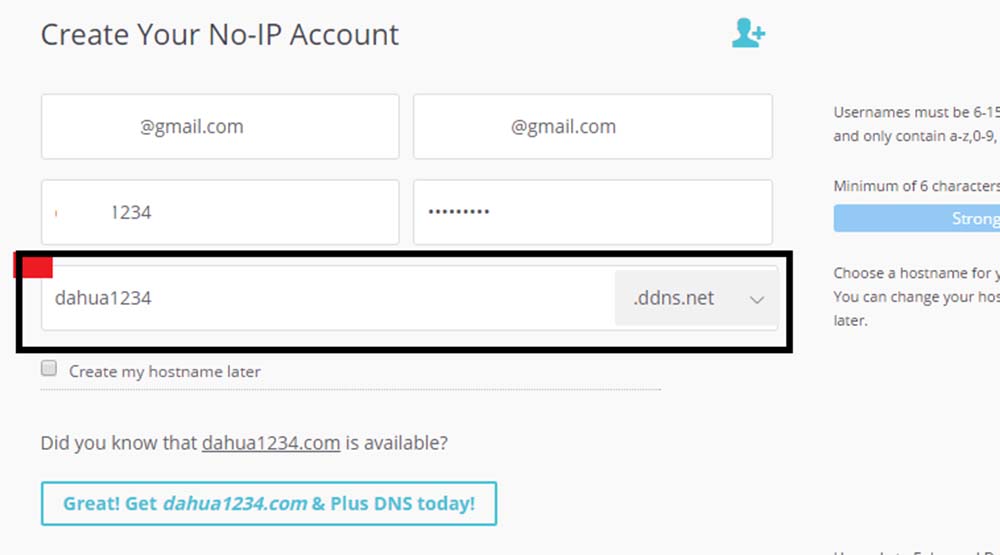The image is a close-up screenshot of a computer screen, displaying a partially visible user interface with a light gray background. Some information on the right-hand side of the screen is cut off due to zooming in. 

In the top left corner, there is the text "Create your Know IP account" next to an icon of a person with a plus sign in turquoise blue. Below this text, there are two rows of rectangular input fields divided into two columns. The top two fields have the text "@gmail.com" inside them. The bottom left field contains the numbers "1234," while the bottom right field displays bullet points, indicating obscured password characters. 

Undeneath these fields, there is a longer rectangular input box with the text "dahua1234" inside it. To the far right of this input box, it says "ddns.net" with a small downward caret for a drop-down menu. This input box is highlighted with a dark black border and a red square in the top left corner.

Below this highlighted section, some additional text is partially visible. Toward the bottom of the screen, there is a turquoise blue rectangle containing the gray text "Get dahua1234.com + DNS today."